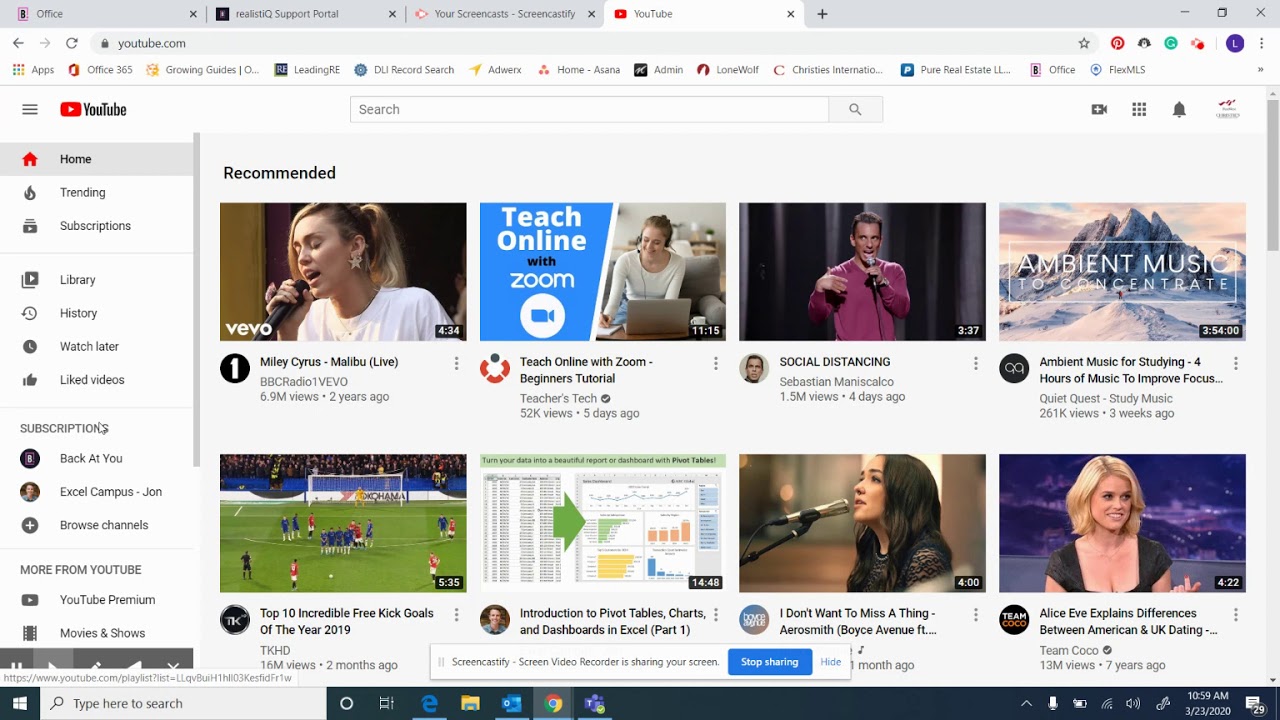This image captures a screenshot of a web browser displaying YouTube. In the address bar, youtube.com is entered, leading to YouTube's home page. A prominent gray bar runs across the top of the page.

On the left sidebar, several categories are listed vertically:
- Home
- Trending
- Subscriptions
- Library
- History
- Watch Later
- Liked Videos

Under the 'Subscriptions' section, specific channels are highlighted, including:
- Back at You
- Excel Campus
- Browse Channels

Additional sections such as "More from YouTube" list:
- YouTube Premium
- Movies and Shows

The main body of the page displays an array of YouTube video thumbnails, each with an associated picture and title:
1. "Miley Cyrus Tech Online with Zoom for Beginners" – likely shows Miley Cyrus or related tech tutorial imagery.
2. "Social Distancing and Sebastian Maniscalco" – features the comedian Sebastian Maniscalco.
3. "Ambient Music to Concentrate" – includes soothing, scenic visuals.
4. "Top Ten Incredible Free Kick Goals of the Year 2019" – showcases dramatic football (soccer) moments.
5. "Introduction to Pivot Tables, Charts, and Dashboards" – displays graphs and charts.
6. "I Don't Want to Miss a Thing by Aerosmith" – possibly includes concert footage or a music video still, showing a person singing.
7. "Alice Eve Explains Differences Between American and UK Dating" – features an image of actress Alice Eve with blonde hair.